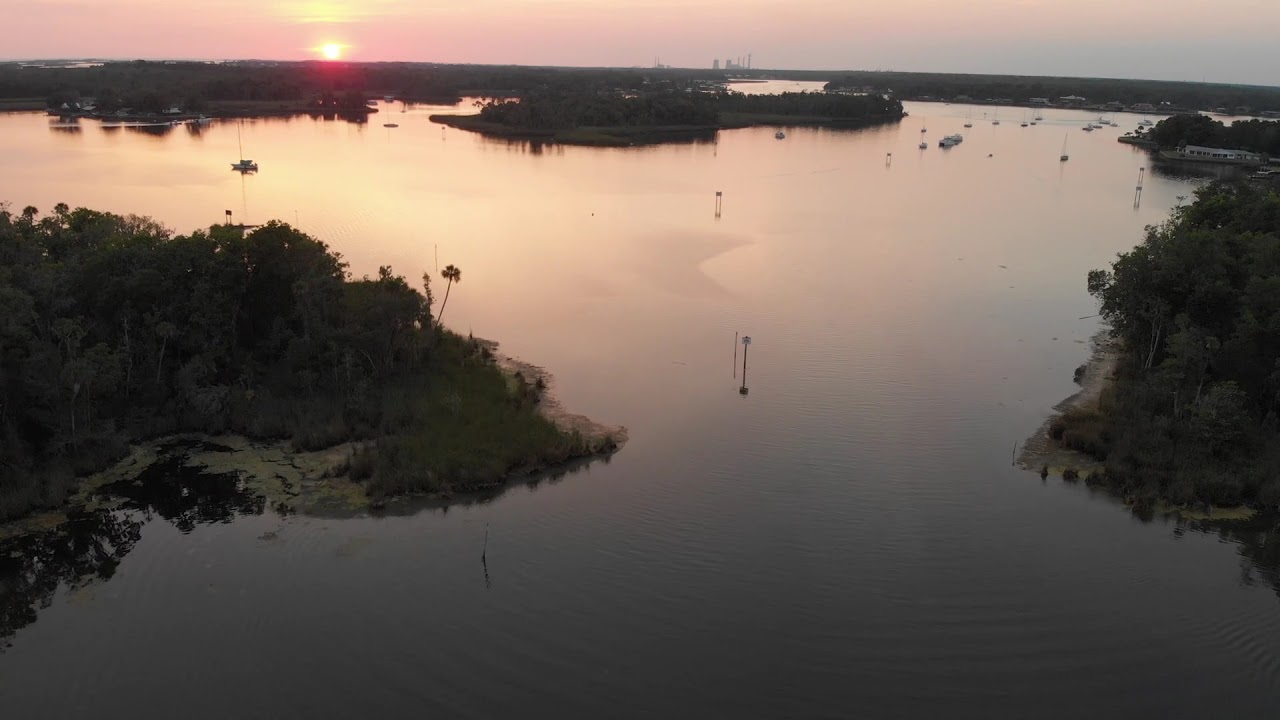This image, taken outdoors during the daytime at dusk, portrays a serene and calm lake or river with the sun setting in the background. The water, smooth and dark, transitions from an orangey-peachy hue near the horizon to a very dark gray closer to the viewer. Gentle ripples, likely caused by distant boats, create subtle textures on the surface. The scene is dotted with small buoys and floating vegetation, giving a somewhat swampy feel. 

The composition includes three notable landmasses: grassy islets at the lower left and right, and a more substantial island in the center. These sections of land are heavily forested, with the trees appearing almost black and gray due to the twilight lighting. An uneven tree line is visible in the distance, providing a natural boundary to the water.

The sky occupies the upper eighth of the frame, painted in shades of pink, orange, and gray around the setting sun, while deeper blue tones persist on the periphery. Overall, the landscape exhibits a tranquil, undeveloped charm, with no houses in sight, and hints of human activity evidenced by the buoys and distant boats.